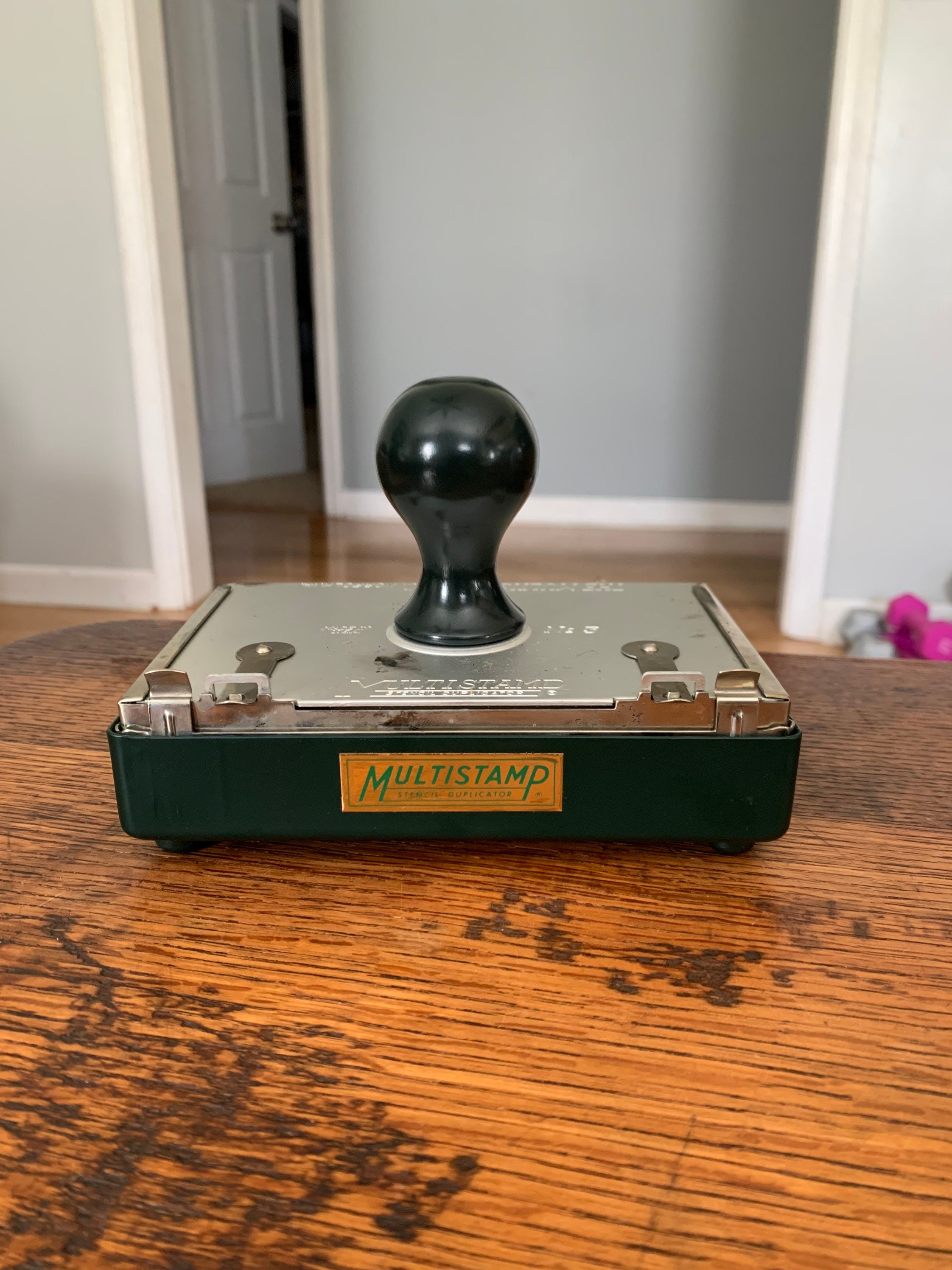The image depicts a color photograph taken in a brightly lit, vacant room with no visible furniture. The main subject is a stamper placed on a shiny wooden table, standing on a brown wooden floor. The stamper has a rectangular box shape with a green base, a silver metal top, and a black, ball-shaped handle resembling a doorknob. The front of the stamper features the words "multi-stamp" engraved in green on a brown sign. The background reveals a gray wall with white trim and a white door that is wide open, likely leading to another room, possibly a bedroom. Black strings adorn an old-looking brown window. Additionally, small dumbbells in gray and pink hues can be seen leaning against the wall on the right side of the image.